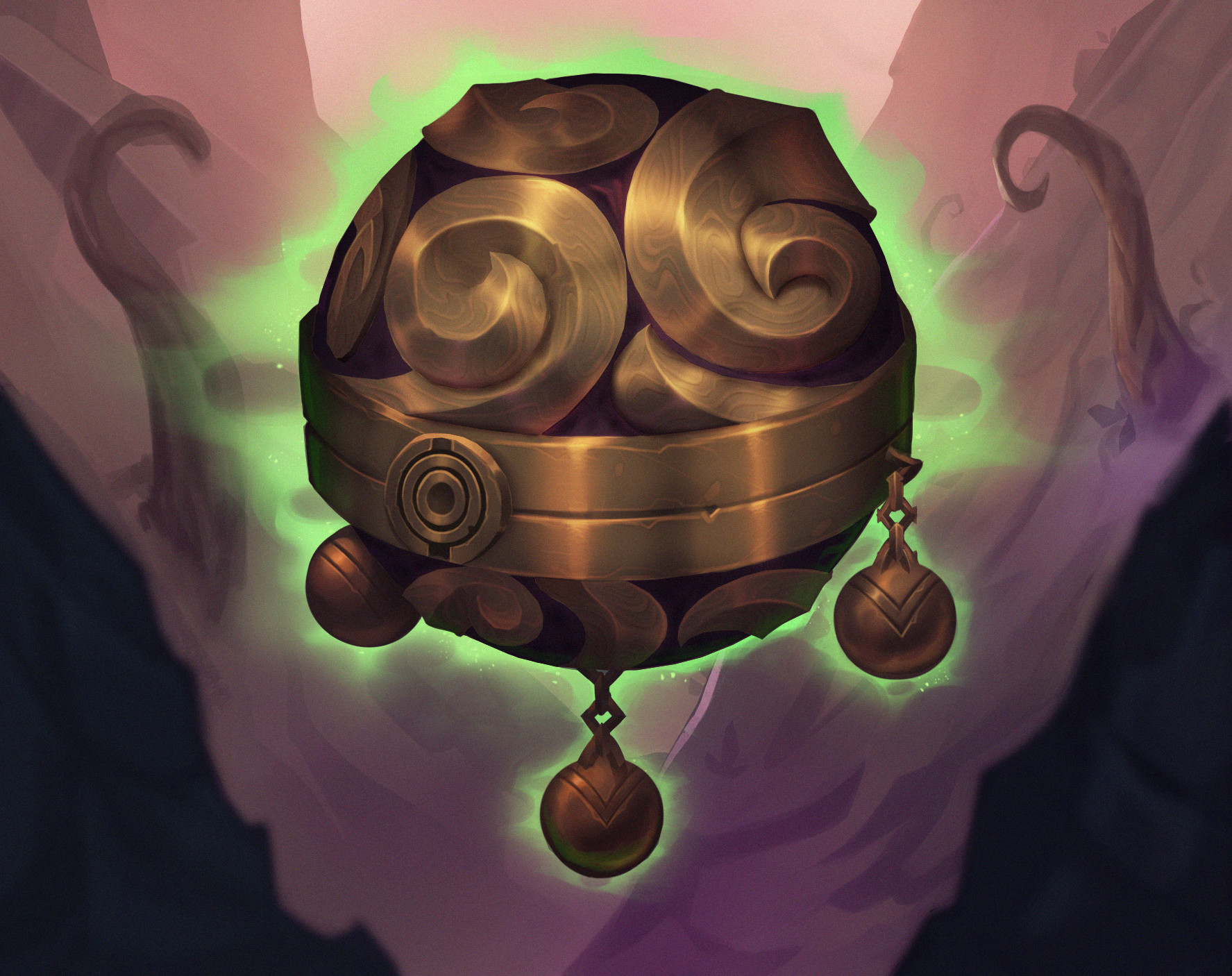The image depicts a vibrant, graphic artwork of a floating, spherical artifact set against a striking, multi-colored background. The artifact is centrally positioned within a rectangular frame, its top and bottom sides longer than its left and right edges. The object itself is circular with a rich reddish body adorned by golden spirals and two prominent gold bands running around its midsection, interconnected at a central circle. Small bronze chains with round balls dangle delicately from its sides and from the bottom. The artifact seems enveloped in a green, smoky halo, creating a glowing effect. The background illustrates a stark contrast: the lower left and lower right corners are dominated by solid black and dark gray hues, while the upper left and upper right transition into blends of pink and purple, cascading down in a wide V-shape. Darker streaks of purple punctuate this gradient. The entire scene is set within what appears to be a valley, framed by stone walls with curling roots emerging from them. The overall surreal and mystical ambiance is underscored by the artifact's ethereal floatation and the luminous green backdrop.